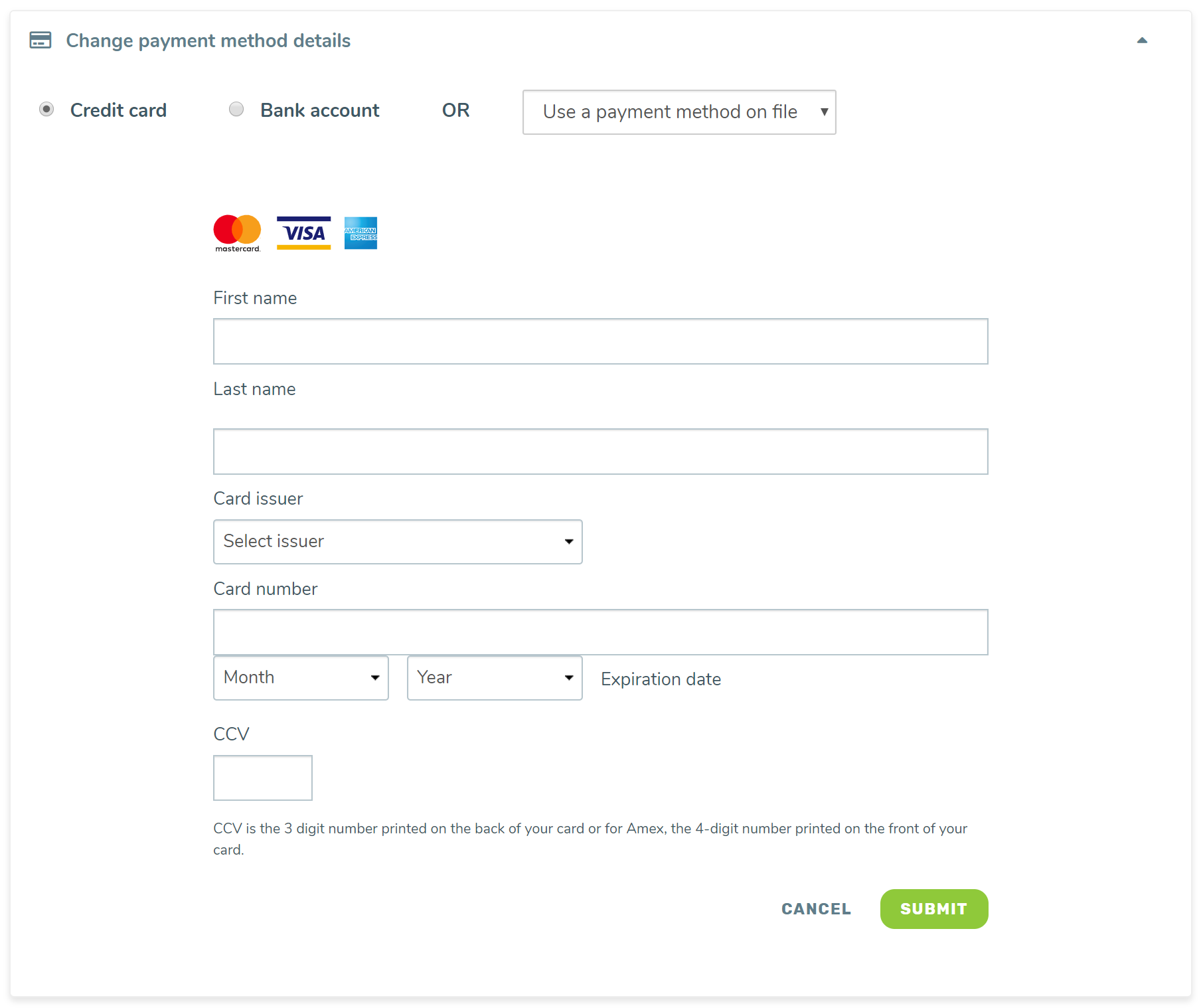**Detailed Caption for Credit Card Payment Landing Page:**

The image depicts a credit card payment landing page. At the top left corner, there is an option labeled "Change Payment Method Details," accompanied by a card symbol. Directly below this option, the default payment method is shown as a selected credit card. To the right of the selected credit card, there is an option to choose a bank account, which is currently not selected. Adjacent to the bank account option, the word "or" is displayed. Further to the right, there is a small box labeled "Use Payment Method on File."

Below this section, the logos of MasterCard, Visa, and American Express are displayed, indicating accepted payment types. The form includes several fields for user input, starting with a "First Name" box followed by a "Last Name" box. Below the name fields, there is a drop-down menu labeled "Card Issuer" with the instruction to "Select Issuer."

Continuing down the form, there is a "Card Number" box that requires the user to input their card details, including fields for the "Expiration Date" with separate boxes for the month and year. Below the expiration date, there is a box for the "CCV Code," with instructions clarifying that this is the three-digit number printed on the back of most cards and the four-digit number on the front of American Express cards.

At the bottom of the page, there are two buttons: a "Cancel" button, which has no color, and a "Submit" button, which is highlighted in green. The overall design of the page maintains a clean, minimalistic appearance with a white background and black lettering, apart from the logos and the green "Submit" button.